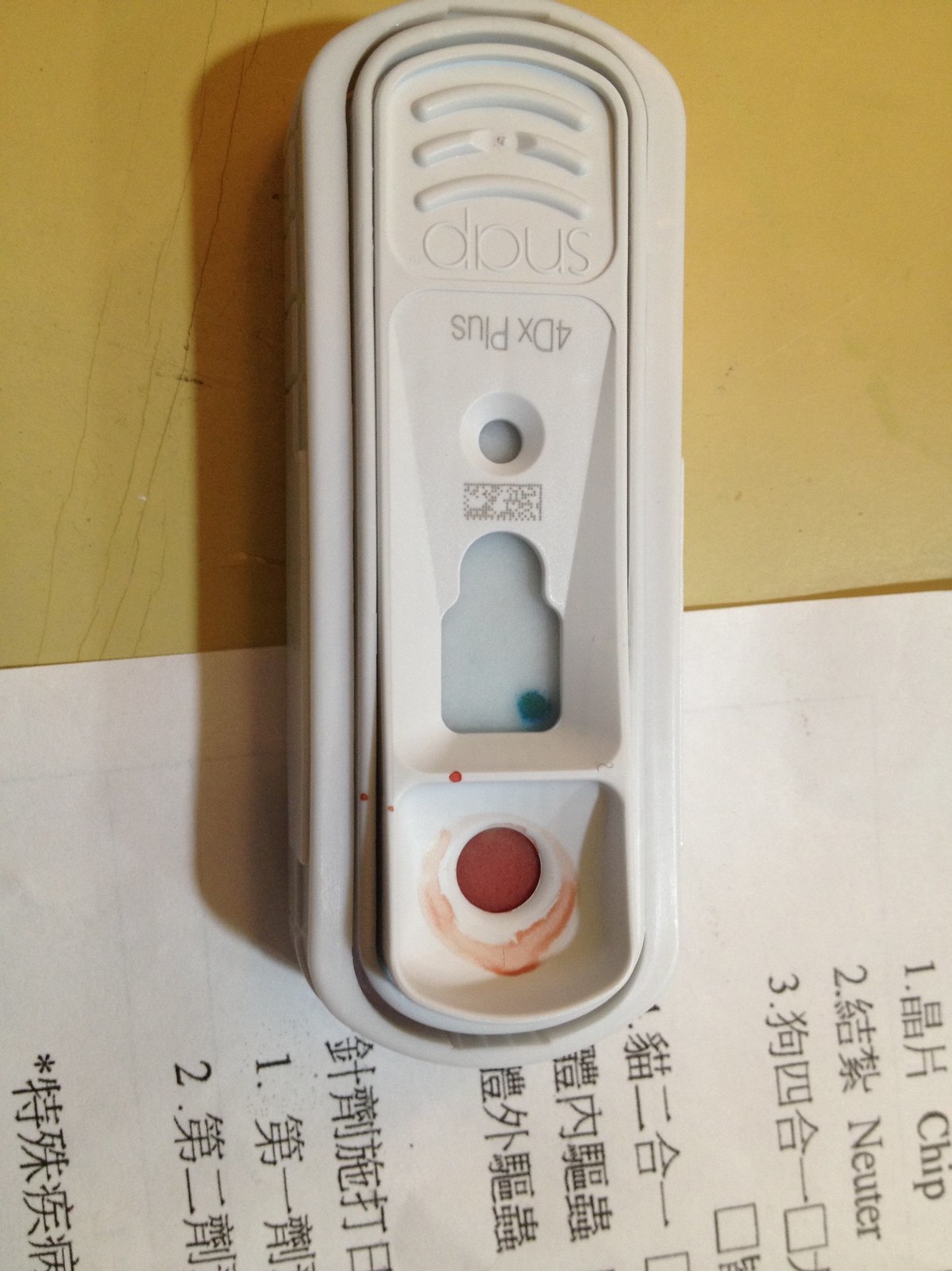This photograph showcases a medical testing device with a design reminiscent of a pregnancy test, though its specific purpose remains unclear. The device is made of white plastic and has an oblong, oval-like shape. Positioned upside down, the device displays the brand name "SNAP" prominently on its surface. Below the logo, there are ridges followed by some text that reads "Dx+P."

The device features three distinct windows. The first is circular, the second has a shape resembling a baby bottle, and the third is also circular. Notably, the bottom circular window appears to be soaked in red, indicative of blood, with some blood visible outside the window as well.

The device rests on a white piece of paper covered in black, typed text. Among the text, a few English words such as "chip" and "neuter" are discernible. However, the majority of the writing appears to be in Chinese characters.